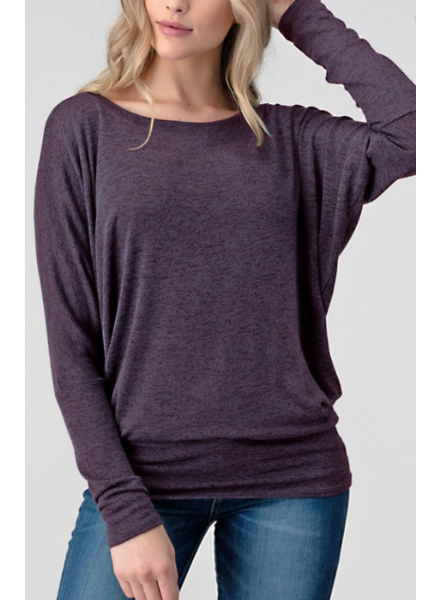In this product image, a blonde-haired female model with shoulder-length hair and pink lipstick is showcasing a purple sweatshirt, which is the focal point of the composition. She is standing against a plain white background, ensuring there are no distractions from the garment. The photograph captures her from just below the nose to above the knees, emphasizing the featured apparel. 

The model's left hand is placed behind her head, gently stroking her hair, while her right arm is crossed in front of her body, contributing to a relaxed and natural pose. She dons a pair of distressed blue denim jeans that fit snugly, contrasting with the loose-fit, lightweight sweater. The sweatshirt, characterized by its darker purple hue and subtle texture with speckles, features a wide neckline and long sleeves that drape loosely around the armpits before fitting snugly at the cuffs and waist. The garment extends just over her hips, combining a baggy yet form-fitting silhouette that accentuates the casual, stylish appeal of the piece.